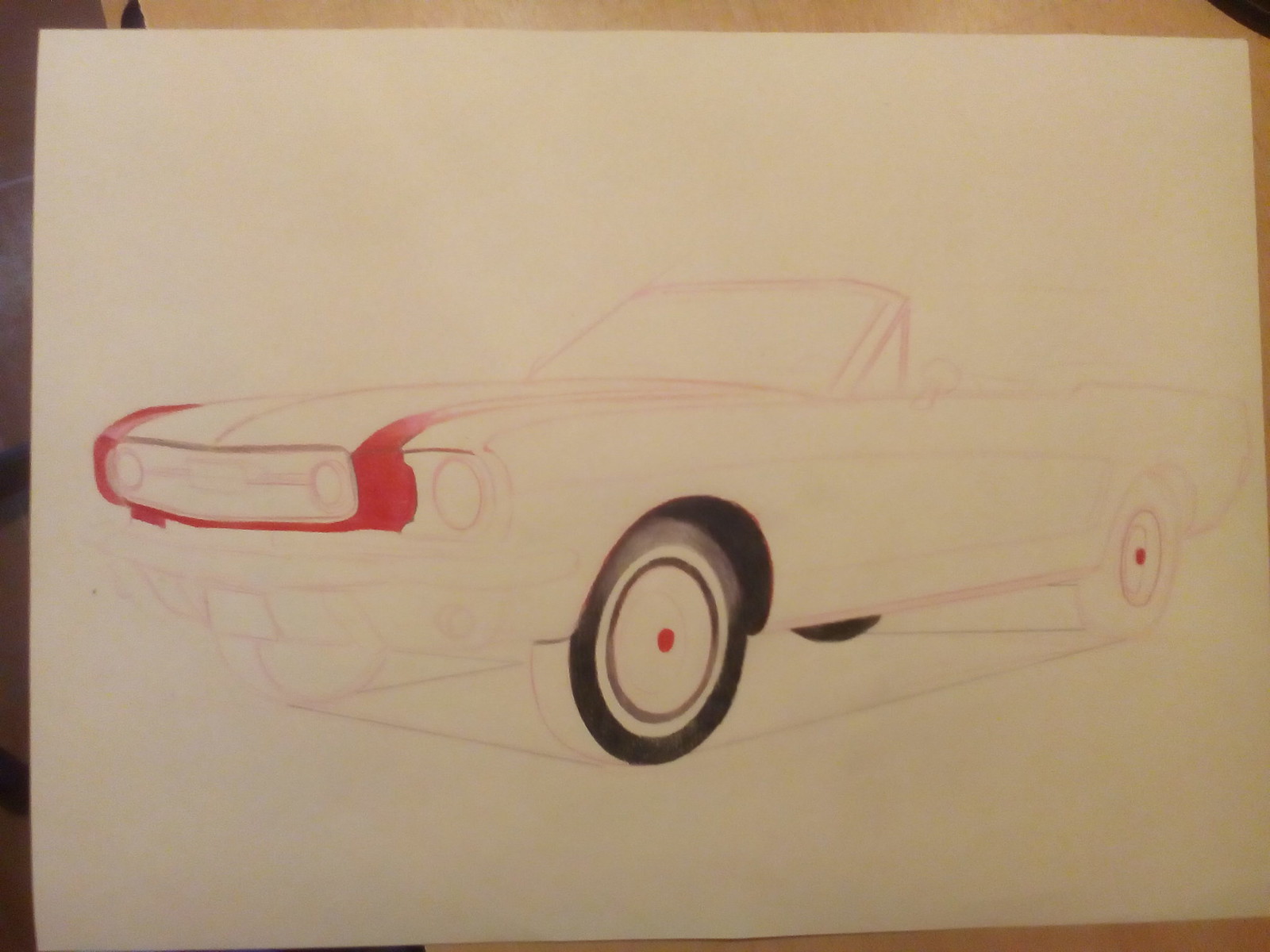The image is an incomplete illustration of a vintage car, likely from the 1950s, crafted with colored pencils, primarily in a red hue. This convertible car, which lacks a roof and prominently features a windshield, is set against a plain white sheet of paper. The illustration reveals intricate details such as a small side mirror and large, elevated tires. The front left tire is depicted in black, accentuated with a red dot at its center, and the rear tire, partially visible, is also black. The artwork rests on what appears to be a wooden table, adding a rustic touch to the scene.